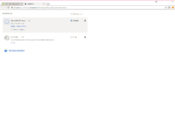The image appears to be a faint screenshot of a user interface, likely from a digital application. At the very top, there's a horizontal red line. Below this, in the upper left-hand corner, there's black text set against a gray background. Underneath this text is a section that looks like it contains an icon and some text, followed by a search bar. The background of the remaining portion of the image is white.

Directly below the top bar, there's black text on the left. Adjacent to this text is a horizontal gray rectangle, within which lies an icon in the upper left-hand corner. To the right of this icon, there are about four or five lines of text. On the far right of this section, there's a bolded word accompanied by an icon.

Moving further down the image, there's a similar setup to the previous gray section, but this one has a white background and one fewer line of text. This section also features a word on the right that is not bolded and includes an accompanying icon. Approximately three lines below this, there's a blue icon with some text written in blue to its right. Due to the faintness of the screenshot, the specific details of the text and icons are difficult to discern.